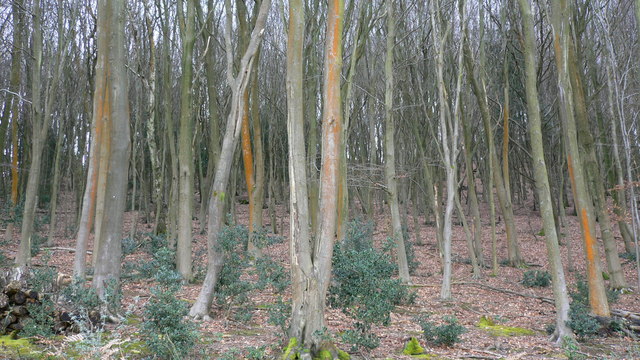This color photograph captures a dense, serene forest filled with numerous vertical tree trunks varying in bark color from pink to gray. The trees are predominantly bare, with only a few small branches sticking out, giving an impression of a forest in late autumn or early winter. The forest floor is covered with a pinkish-gray litter of loose leaves and rough ground, scattered with dead gray sticks. Among this litter, patches of green shrubbery and brush are visible, adding texture to the scene. On the left side of the image, a small pile of logs is surrounded by small green bushes, with light green moss growing at the base of some trees. The background features a dense cluster of trees with glimpses of a blue, lightly-clouded sky. The image is a horizontal rectangle, with predominantly earthy and muted tones, capturing the natural, undisturbed beauty of an outdoor woodland setting.